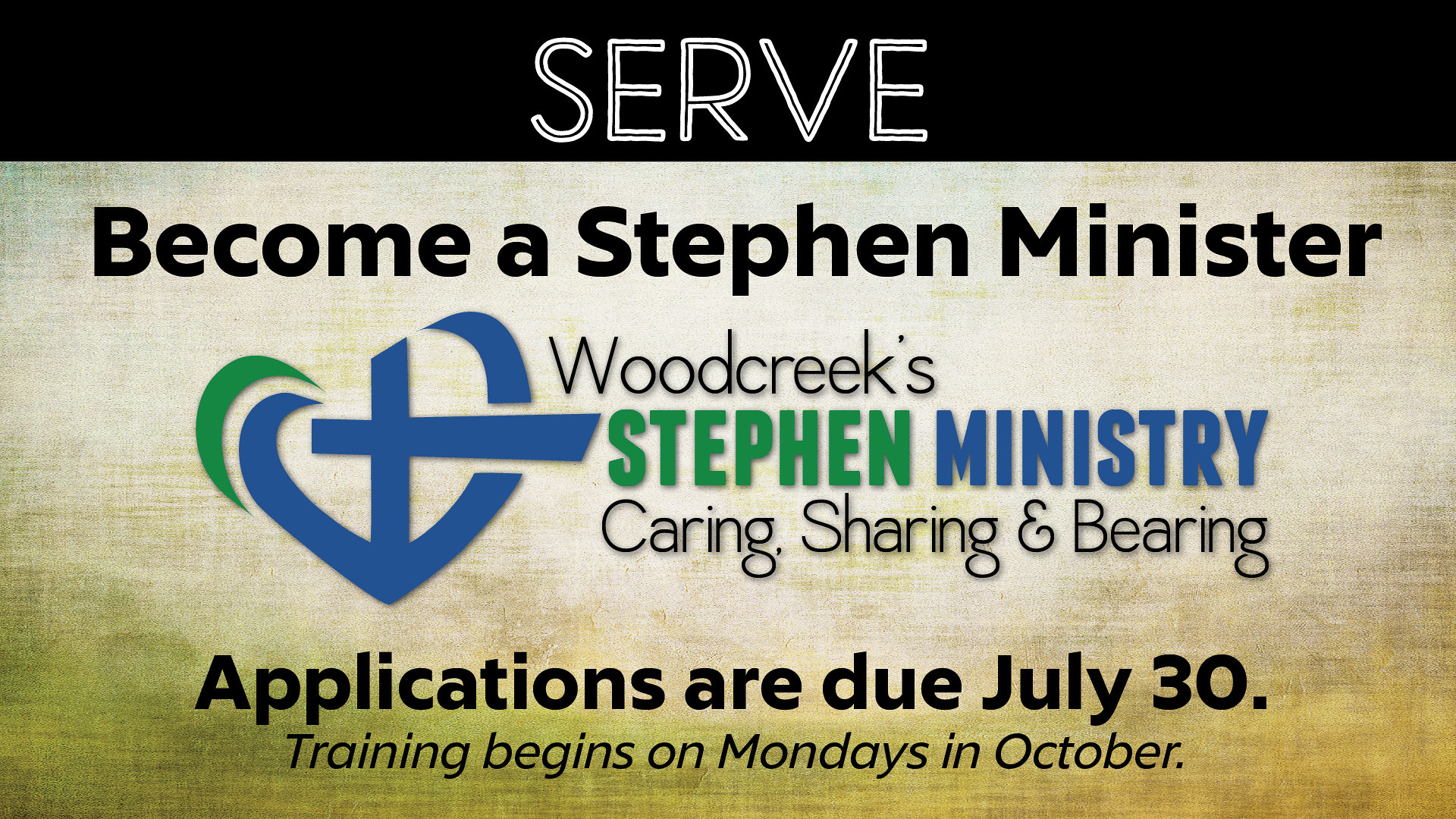This digital poster, in landscape orientation, begins with a thick horizontal black strip at the top. Centrally positioned within the strip, the term "SERN" appears in prominent white text. Directly below this strip, the text reads, "Become a Stephen Minister." In the left section below, a logo features a three-quarters heart with a cross extending out to the right. Adjacent to this logo, the text "Woodcreek's" is displayed, followed by "Stephen Ministry" split into "Stephen" in green and "Ministry" in blue. Below this, the slogan "Caring, Sharing, and Bearing" appears in black lettering. Further down, the text specifies that "Applications are due July 30" and beneath that, in smaller text, "Training begins on Mondays in October." The image has a nuanced background transitioning from shades of tan and brown, lending a subtle yet professional feel. This digital poster likely serves as an advertisement or informational card aimed at recruiting for the Stephen Ministry, and its polished design suggests a religious or community-oriented purpose.